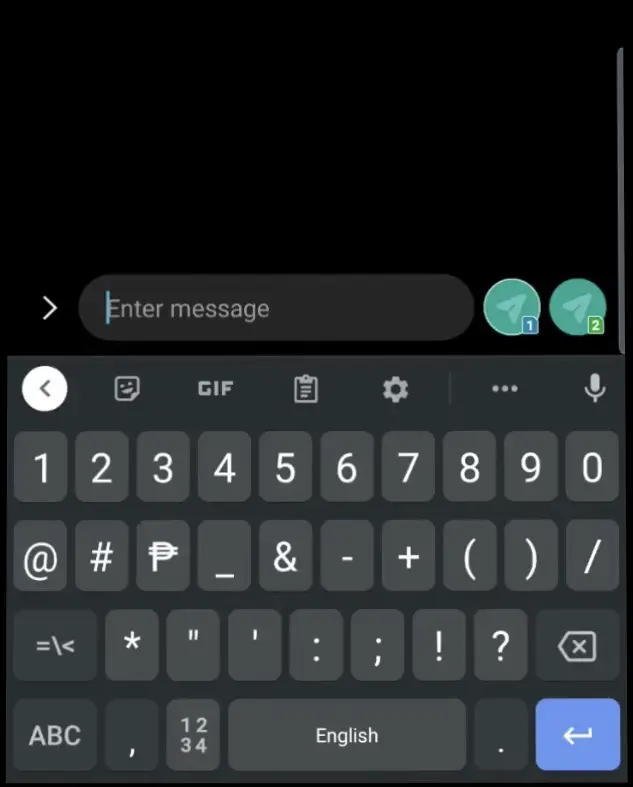This image captures a dark gray and black virtual typewriter keyboard on a computer screen, accented with lighter gray keys featuring white letters and numbers. The keyboard is currently set to the numbers and symbols page. At the top of the interface, a sticky note icon with a face is displayed, followed by icons for GIFs, a noteboard, settings, a three-dot menu, and a microphone on the far right.

The keys include numbers one through zero, special characters like the pound sign (#), and symbols such as an at sign (@), a currency symbol (₹), underscore (_), dash (-), plus (+), open and close parentheses (()), forward slash (/), equals (=), backward slash (\), less than (<), asterisk (*), double quotes ("), single quote ('), colon (:), semicolon (;), exclamation point (!), and question mark (?). The backspace key is present as well.

Below these keys, options for toggling the keyboard are provided: ABC for letters, a numeric cluster (1234), a space bar labeled "English," a period (.), and a left-pointing arrow key for backspace. Directly above the keyboard, the phrase "Enter message here" is displayed, leaving space for text input.

On the right side of the screen, there are two small, green circular indicators labeled "1" and "2". The rest of the screen surrounding the keyboard is black, providing a stark contrast that helps the keyboard stand out.